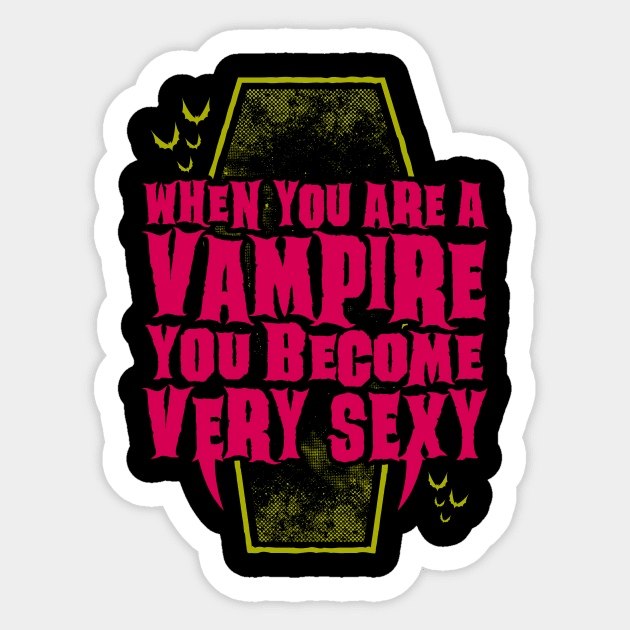This image features a square sticker, approximately 4 inches in height and 3-4 inches wide, against a light gray background. The sticker's irregular shape has a white border and an inner black outline. Central to the design is a simplified gold line drawing of a traditional six-sided coffin with pixelated gold shading on its black background. Surrounding the coffin, there’s an inscription in bold red font stating, "When you are a vampire, you become very sexy." Notably, the 'E' in "very" and the 'X' in "sexy" have fangs extending from them, enhancing the gothic appeal. In the upper left and lower right corners of the sticker, there are small gold bat illustrations, adding to the vampiric theme. The overall atmosphere suggested by the elements and colors used in the sticker is both gothic and comic-like.